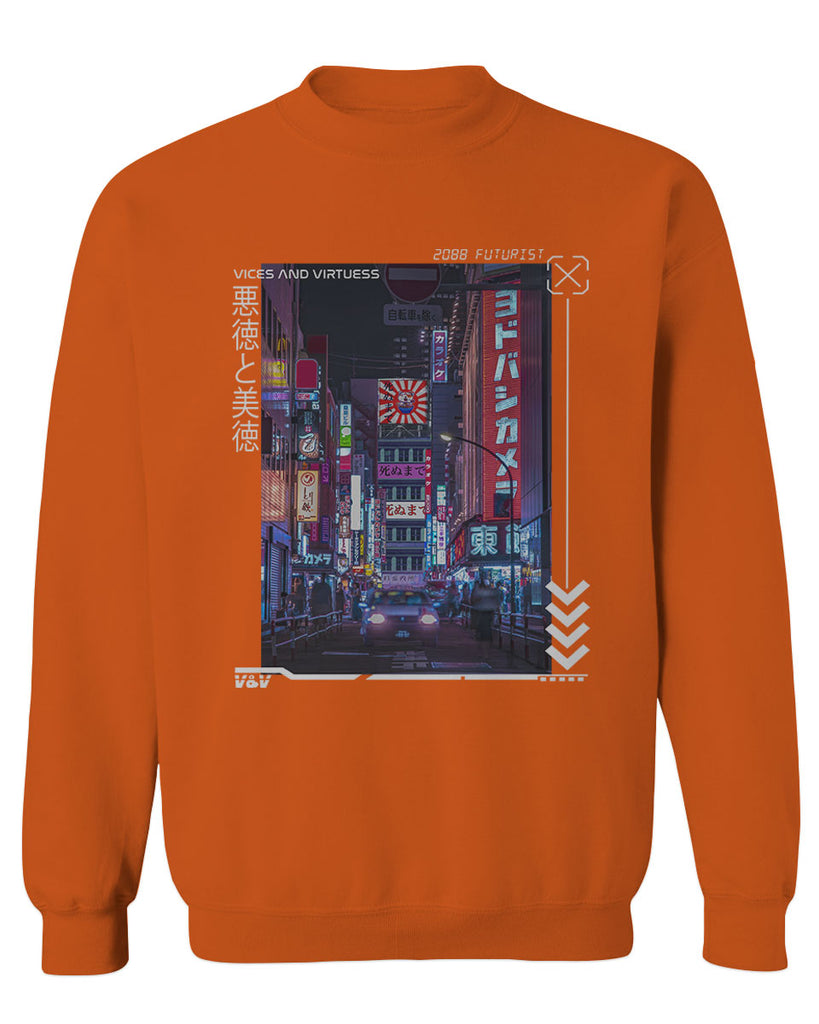This is an image of an orange sweater against a white background, prominently displaying a cyberpunk-style artwork on the front center. The artwork depicts a futuristic night scene of a busy Japanese city, likely Tokyo. At the forefront, a car faces head-on, surrounded by sidewalks filled with people. The scene resembles a vibrant, illuminated cityscape akin to Times Square, with buildings adorned with bright Japanese signs on the left, right, and center.

In the artwork’s top right corner, "2088 Futurist" is written with an 'X' above four downward-pointing arrows and a line extending from it, reminiscent of a clickable computer interface. Adjacent to this on the left, the text "Of Vices and Virtues" is displayed, with additional vertical Japanese text positioned further left. On the bottom left of the artwork, the initials "VNV" are inscribed in white. Overall, the sweater combines elements of futuristic design with neon-lit urban imagery, encapsulating a vision of Tokyo in the year 2088.